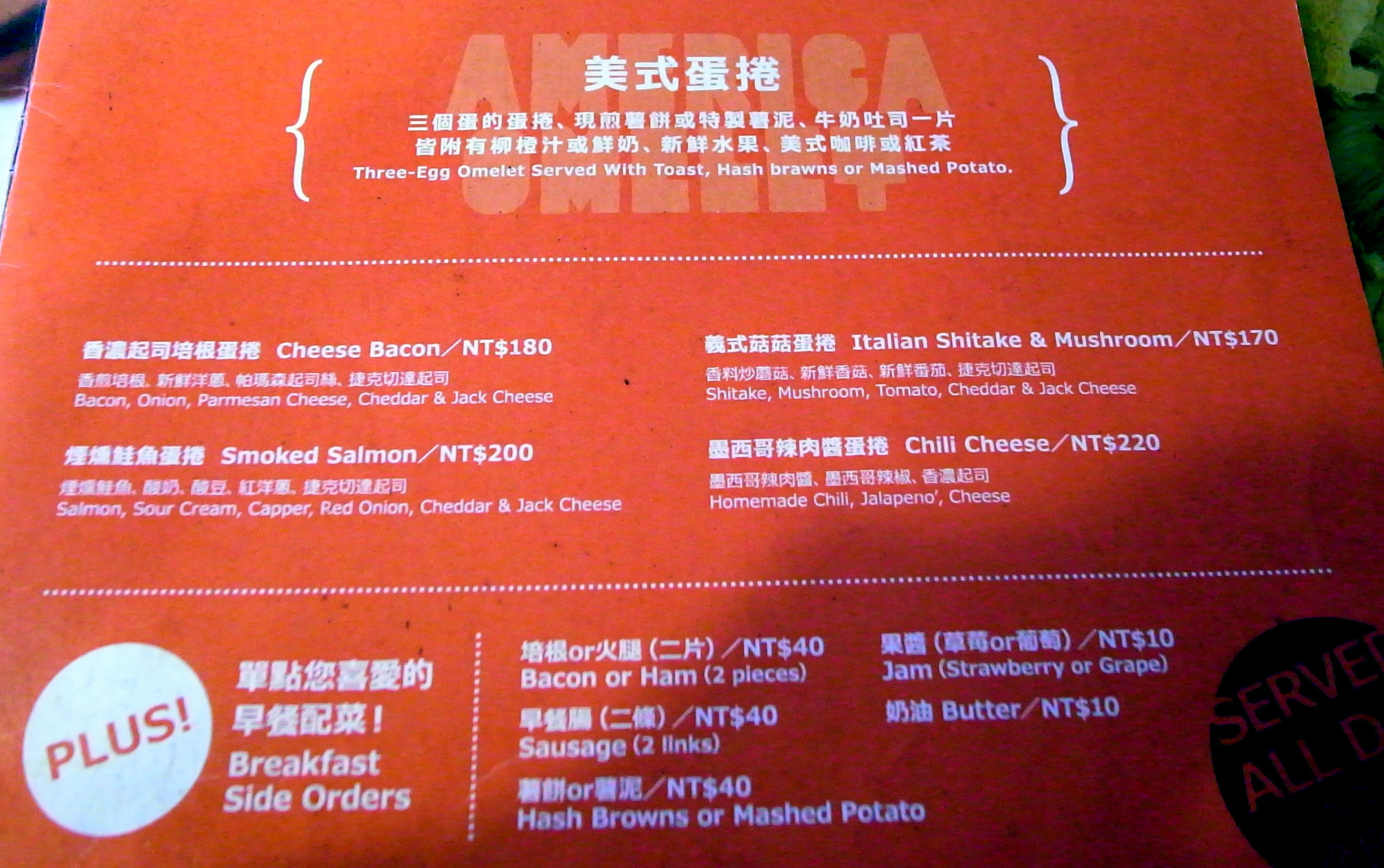The image showcases a rectangular menu, approximately 30% wider than it is tall. It appears to be placed outdoors or indoors, though the setting isn't explicitly clear. The menu is predominantly red, with a medium hue that spans from left to right, subtly fading at the edges in the upper corners.

At the top, the menu features text in an Asian script, likely Chinese characters, followed by corresponding English translations in white text. The menu is organized into four distinct sections:

1. The top third of the image highlights the primary offering: a three-egg omelet served with a choice of toast, hash browns, or mashed potatoes.
2. The second third lists variations of the omelet, including:
   - Cheese and bacon
   - Smoked salmon
   - Italian shiitake and mushroom
   - Chili cheese
3. The bottom third of the menu is split, with the left portion detailing "Breakfast Side Orders" beneath a red "plus" sign within a white-shaded circle. Side options include:
   - Bacon or ham
   - Sausage
   - Hash browns or mashed potatoes
   - Butter or jam

The entire presentation is characterized by a clear, structured layout, making it easy to navigate the various breakfast choices and accompanying side orders.